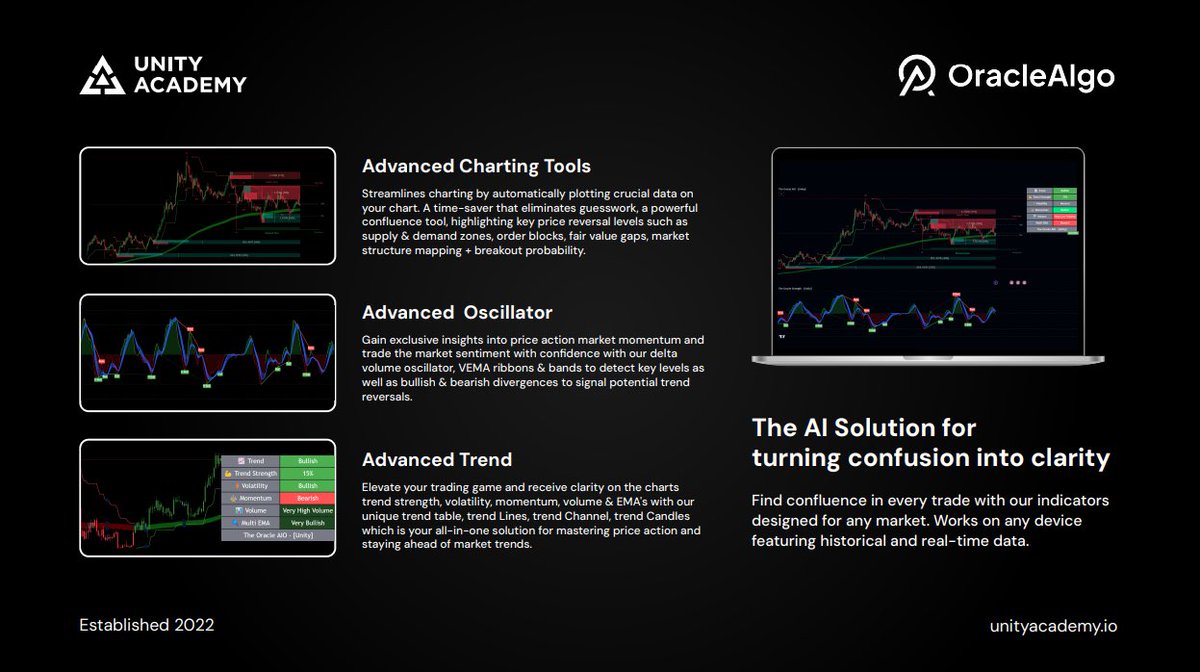The image is a sleek, visually compelling advertisement for the website UnityAcademy.io, established in 2022. It prominently features the Unity Academy logo in the top left corner and the Oracle Algo logo in the top right corner. The advertisement leverages a black background with white text, enhanced by diverse graphs in vibrant colors ranging from purple and blue to green and red. Centrally placed visual content includes three main types of advanced charting tools: advanced charting tools, advanced oscillator tools, and advanced trend tools. 

Each graph is surrounded by explanatory text. For instance, advanced charting tools are described as a time-saving feature that automatically plots crucial data on your chart, highlighting key price reversal levels like supply and demand zones, and order blocks. Advanced oscillators provide exclusive insights into price action and market momentum, using Delta volume, VEMA ribbons, and bands to detect critical levels and signal potential trend reversals. Advanced trend tools aim to clarify chart trends by analyzing trend strength, volatility, and volume with unique trend tables, lines, and channels.

Additionally, a laptop outline houses many of the graphs and symbols, correlating to the broader theme of AI solutions designed to turn confusion into clarity. The pitch highlights the benefits of their tools, like eliminating guesswork and mastering price action across any market and device, using both historical and real-time data.

The ad's bottom left corner marks the establishment year '2022,’ while the bottom right corner lists the website 'UnityAcademy.io'. This comprehensive and visually appealing advertisement effectively communicates the functionalities and benefits of the advanced charting tools offered by Unity Academy and Oracle Algo.